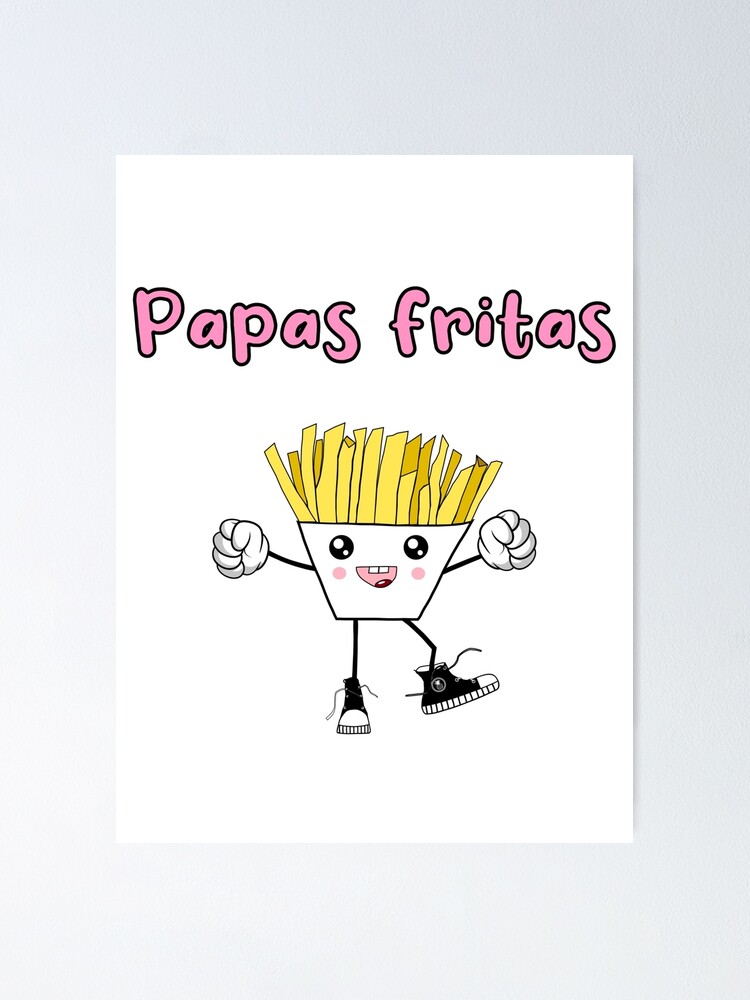This is a hand-drawn cartoon illustration set against a light gray background with a white rectangle in the center. Within this rectangle, an upside-down white trapezoid represents a playful, anthropomorphized container of pale yellow French fries, resembling hair. The container's face features two black eyes with white dots, pink circles for cheeks, and an upside-down pink half-moon mouth displaying two white top teeth and a dark red tongue. The character, exhibiting lively movement, has skinny black arms, each ending in large white gloves with clenched fists raised high, and legs adorned with classic black Converse shoes with white toes. One foot is planted firmly on the ground, while the other is lifted, conveying a sense of dancing or jumping. Above the figure, vibrant pink text outlined in black spells out "Papas Fritas." Overall, the illustration exudes a cheerful, whimsical vibe, likely designed as a fun poster, perhaps for a restaurant.